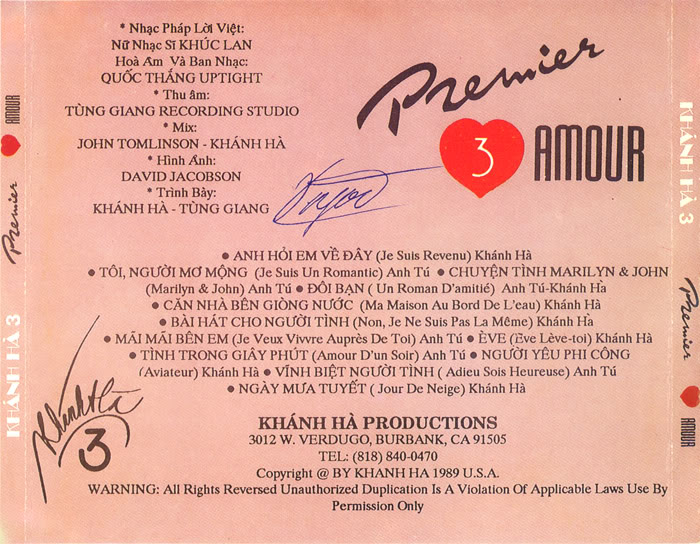The image, likely the insert from a CD case, features a dark pink background adorned with text primarily in French and Vietnamese. Dominating the top is the word "Premier" written diagonally in a bold, black cursive font. Just below it lies a red heart containing a white number "3." To the right of the heart is the word "Amour" in large black text. At the center left, a blue ink signature, complete with cursive and swirled lines, is visible but unreadable. The left side of the image displays a series of black bullet points and accompanying text lines, presumably song titles or performer names, which continue in a structured pattern towards the center. In the lower-left corner, there is another bold black number "3" with an additional black signature above it. At the bottom, "Conha Productions" is prominently labeled above the address "3012 West Verdugo, Burbank, California, 91505," accompanied by a telephone number "818-840-0470." Additional text indicates copyright information from 1989, with a note about all rights reserved and unauthorized duplication.